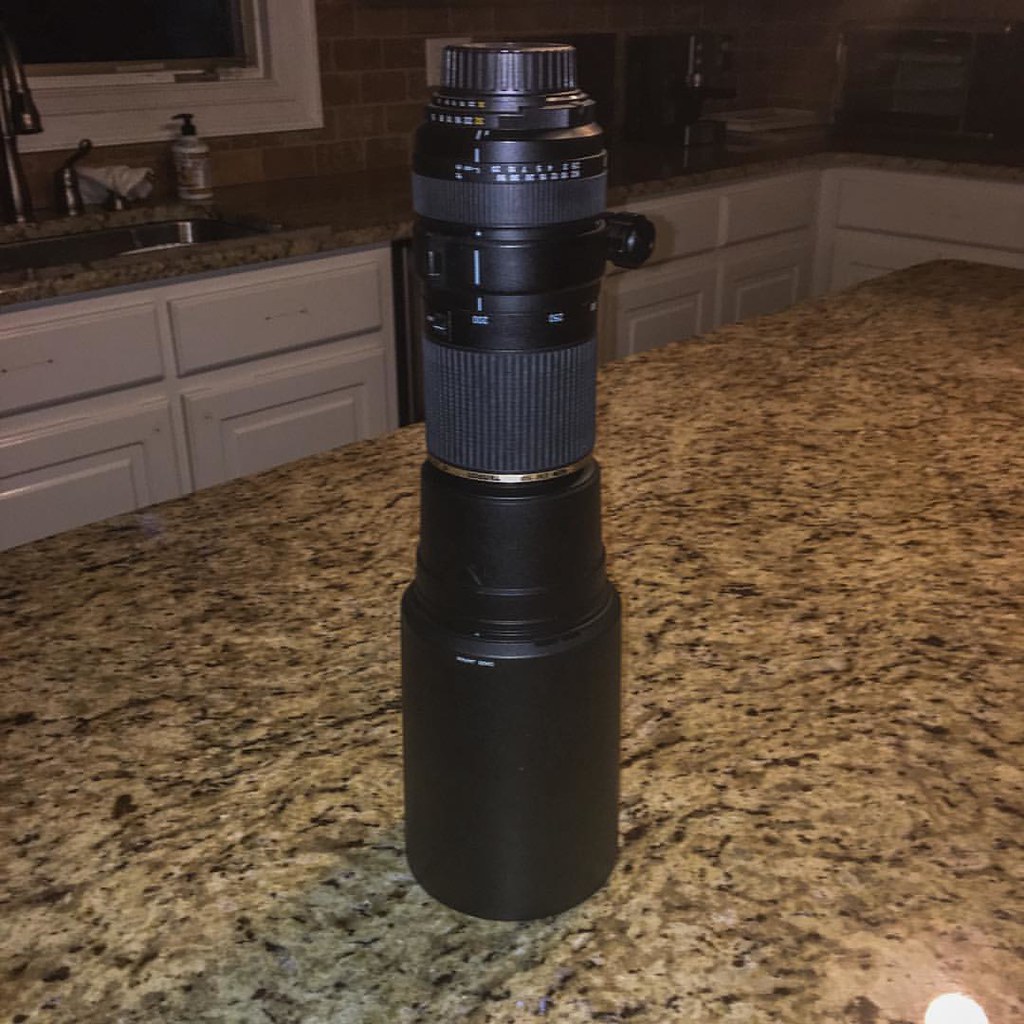This is a detailed photograph of a telephoto camera lens standing upright on a marble kitchen island. Dominating the center of the image, the lens is prominently black with a gold accent line in the middle and features multiple rigid sections with ridges all around. The side of the lens displays measurement settings and white lettering, contrasting against the black exterior. It also includes screws and adjustment mechanisms near the top, and an attachment section that enables it to connect to another barrel. The lens is capped with a protective cover.

The kitchen showcases white cabinet fronts and a granite countertop. In front of a large white wooden frame window with brick-patterned tile walls stands a prominent sink, equipped with a substantial tap and a bottle of hand wash nearby. The room appears dimly lit, which highlights the sleek design and details of the lens.